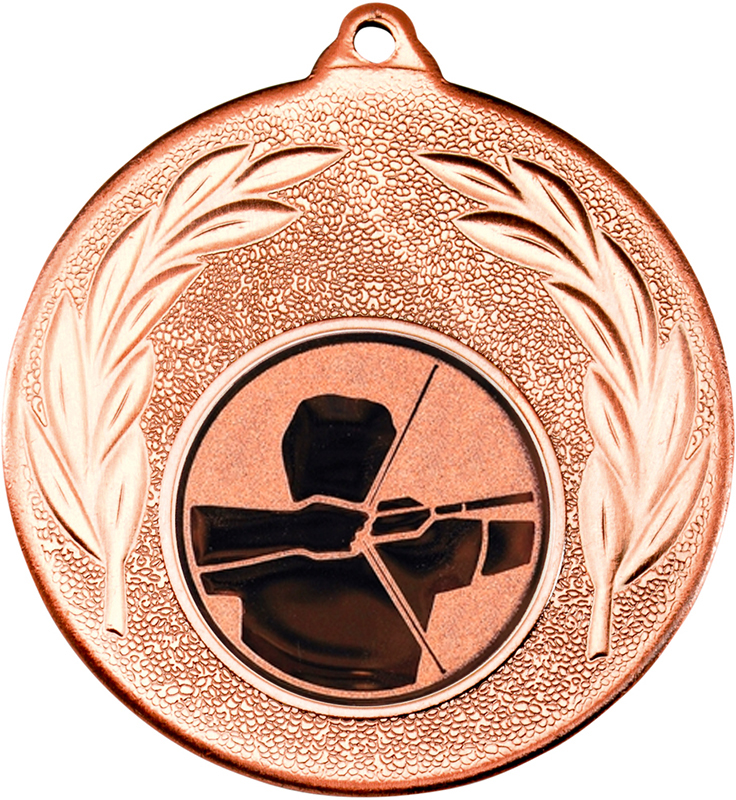This image features a round, textured, bronze-colored medal with an intricate design suitable for being worn as a necklace. At the top of the medal, there is a small protrusion with a hole, designed for a chain to be threaded through. The bronze surface has a textured finish, resembling fish scales, giving it a unique aesthetic. Flanking the bottom-center of the medal are two engraved branches with leaves, adding an elegant touch to the design. The focal point of the medal is a central circular image depicting a stylized, dark figure of an archer in the act of shooting an arrow to the right. This image is set against a copper-colored background and is encircled by a black ring, which is further bordered by a white ring. The overall craftsmanship suggests the medal could be an award, possibly for an archery competition.